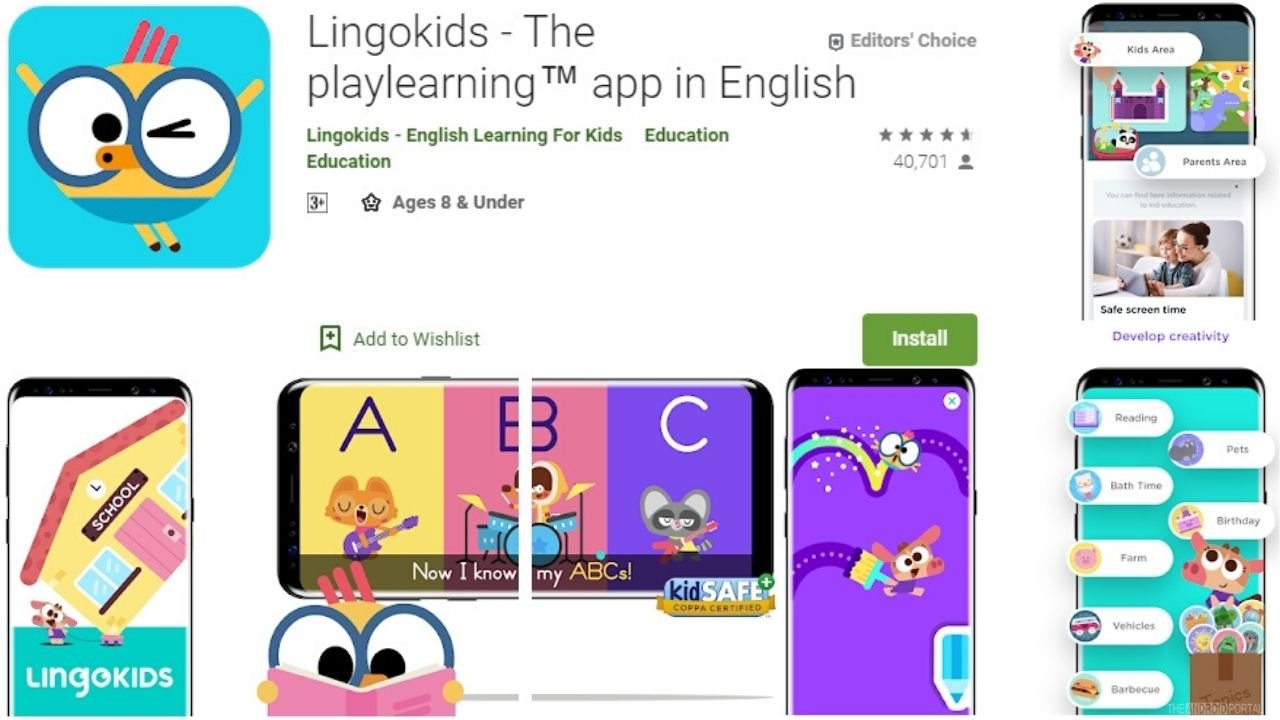This is an advertisement for an educational application called "Lingo Kids: The Play Learning App in English." The app's icon is a blue square featuring a cheerful yellow bird with two large, round eyes—one of which is playfully winking. The bird has its hands and feet raised in the air, signifying excitement and fun, and it sports three small red feathers on its head. 

To the right of the main advertisement, there are screenshots showcasing the app’s user interface, offering a glimpse into its engaging and kid-friendly design. A prominent green rectangular button labeled "Install" invites users to download the app, while an additional option allows for bookmarking the app to a wishlist. "Lingo Kids" is highlighted as an "Editor's Choice," emphasizing its high quality.

The app is recommended for children aged 8 and under and is particularly suitable for kids as young as three years old. Impressively, it has received a rating of 4.5 stars out of 5 from a substantial 40,701 reviewers, reflecting its positive reception and effectiveness as a learning tool.